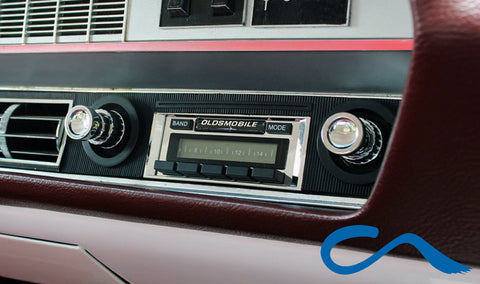The image depicts the interior of an Oldsmobile vehicle, specifically focusing on its classic factory stereo system embedded in a cherry red, possibly leather, dashboard. Centered in this close-up view, the rectangular radio unit features a tape player slot flanked by two distinctive chrome knobs—one on each side. Above the tape slot, the word "Oldsmobile" is prominently displayed, with a band button on the left and a mode button on the right. Below the slot, five black buttons likely intended for various tape operations such as play and rewind are lined up. Surrounding the stereo system and blending into the sleek black dash, chrome accents add a vintage touch. The dashboard also includes air vents positioned to the left of the stereo, and a blue C-shaped logo with a drag mark design in the bottom right corner. A white area beneath this setup suggests the presence of a glove compartment, adding a practical note to the stylish, retro setup.